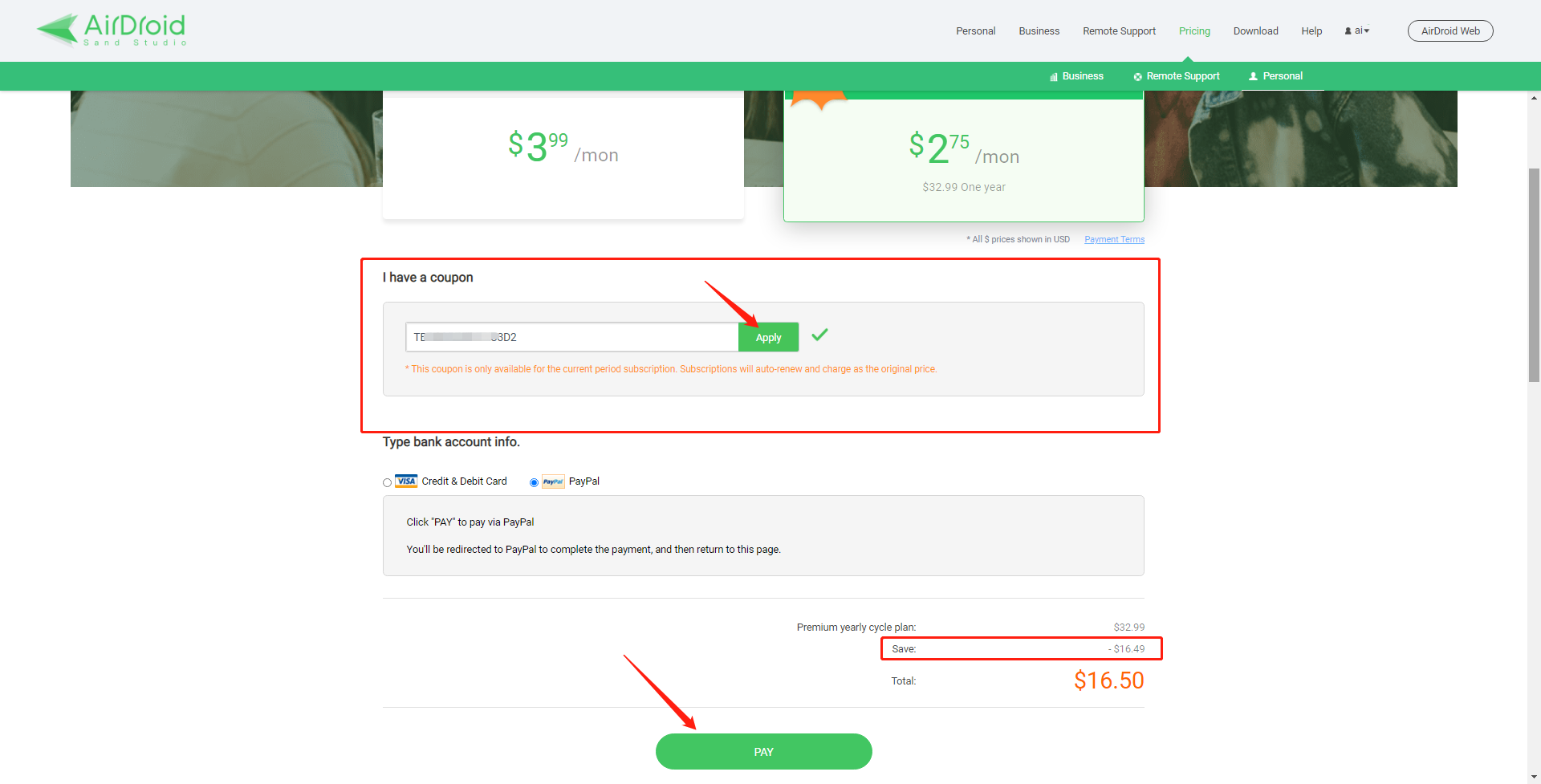The image is a snapshot of a webpage from the website AirDroid. In the top-left corner, "AirDroid" is prominently displayed in green text. Directly beneath this, a horizontal green bar spans the width of the page. To the right of the AirDroid logo and bar are seven menu options, written in black text.

The main content of the page shows a partial screen of what appears to be a checkout or payment interface. A red circle highlights a dialog box labeled "I have a coupon," which features a text entry field where users can input their coupon codes. Beneath this coupon dialog box is another field designated for entering bank details.

A conspicuous green button labeled "Pay" is located below the bank details section. The total amount for the purchase displayed on the screen is $16.50.